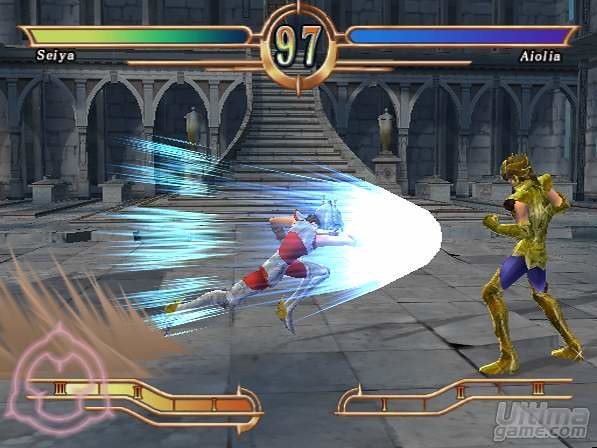This screenshot from a video game resembles a fighting game reminiscent of Mortal Kombat. It features two characters poised for battle against a backdrop dominated by various shades of gray. The left-hand character, named S-E-I-Y-A, is dressed in red and gray and is caught in mid-motion, charging towards the opponent with a whitish-blue flame or light force field emanating in front. Seiya is flanked by a blue light and stands on a gray, square-shaped floor. The right-hand character, named A-I-O-L-I-A, is in a fighting stance, dressed primarily in light green with blue details on their shorts. Above the battleground, atop a gray staircase adorned with urns, arches lead to a second floor out of sight. At the top of the screen, the number 97 is displayed in a gold ring, with bars indicating the energy or life of each player—yellow, green, and blue on the left, and blue and purple on the right. The scene exudes an atmosphere of combat readiness, set within a monochromatic arena.